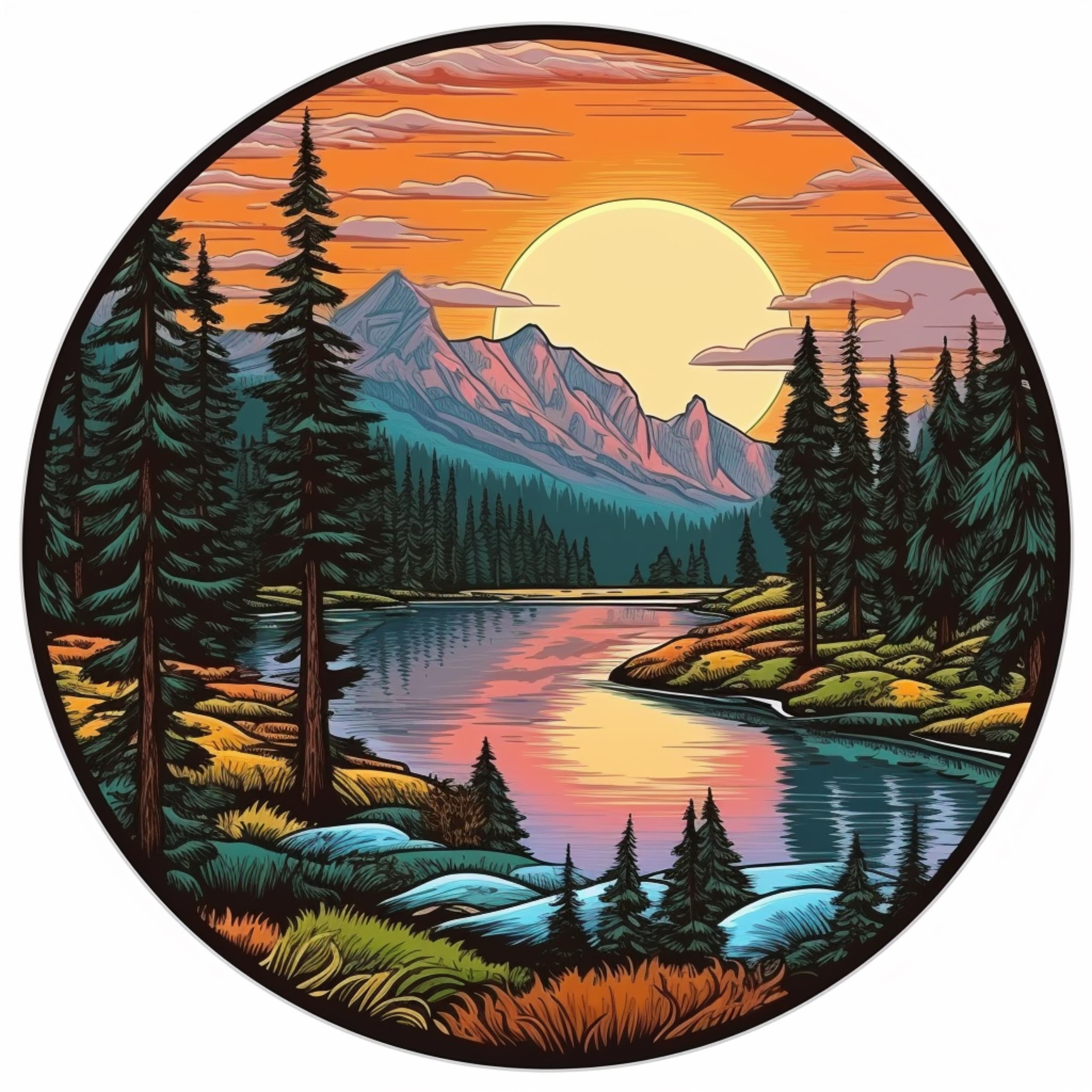This illustration showcases a vibrant and serene mountainous landscape encapsulated within a circle with a bold black outline. At the center, a tranquil river courses through the scene, flanked by lush shorelines adorned with tall, slender pine trees. The river's calm waters reflect the brilliant yellow sun, either rising or setting, casting an enchanting glow over the scene. 

The terrain features a kaleidoscope of colors, with green, red, and yellow hills juxtaposing blue stones, creating a striking visual mosaic. In the background, majestic mountains rise, their lower regions painted in cool blues, transitioning to a pinkish hue as they ascend. Above, the sky blazes in a rich orange, punctuated by ethereal pink clouds, adding to the overall tranquility of the illustration.

Every element, from the serene river to the vibrant color palette, evokes a peaceful and reflective ambiance, reminiscent of the scenic splendor found in the Northwest United States. The meticulous graphic design suggests it could perfectly adorn a product label, perhaps something like trail mix, capturing the essence of nature’s beauty in a single, vivid image.